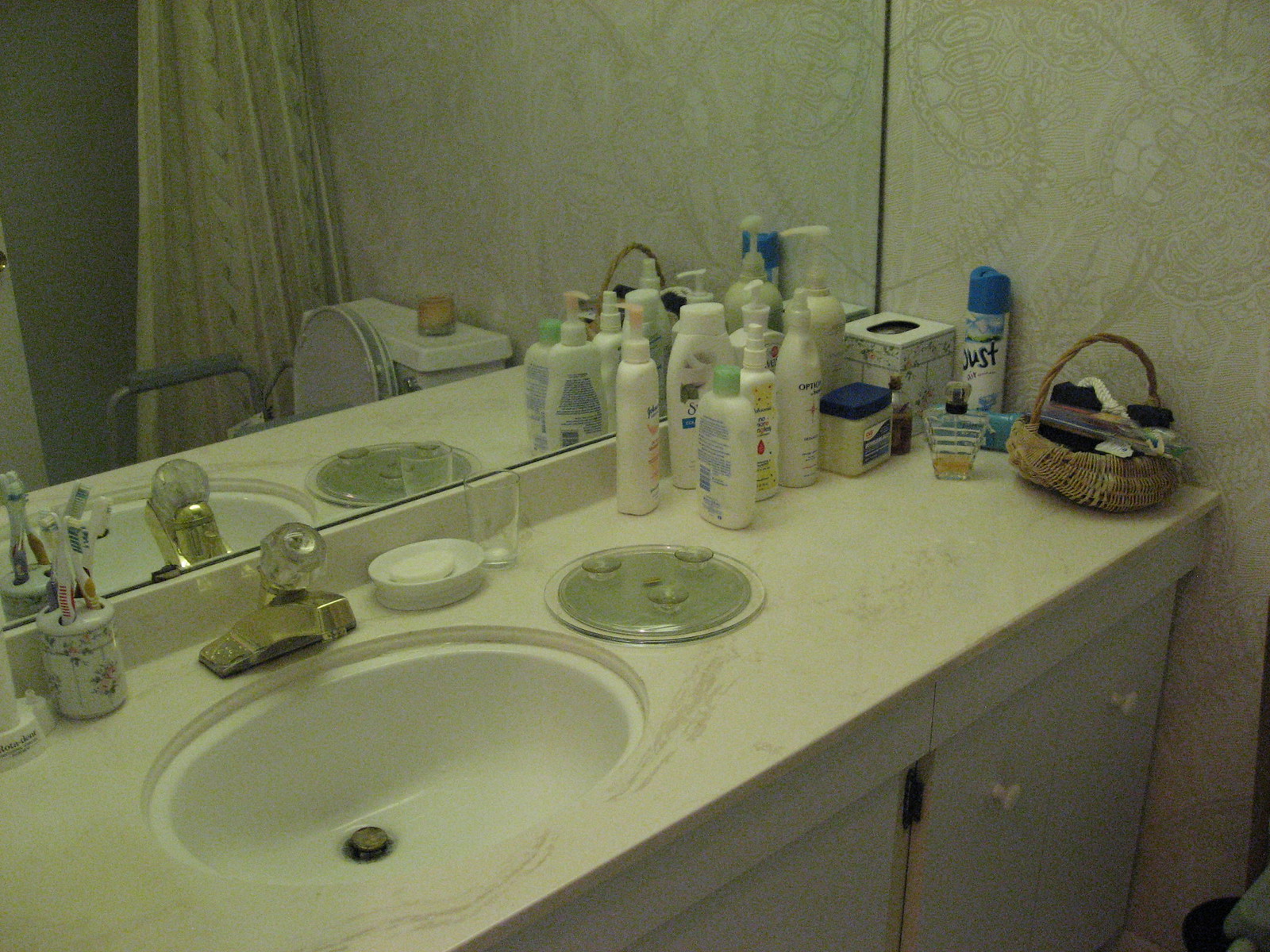The bathroom features a serene atmosphere with its pale green wallpaper adorned with delicate, varying shades of green leaves. Spanning almost the entire length of one wall is a large mirror, reflecting its surroundings. Below the mirror, a light green and white mingled countertop holds various items. Among them is a white statue of a man and woman dancing, accented with small pink flowers at the base. Next to the statue is another small white ornament.

The mirror also shows a white toilet equipped with a handle on the side for assistance, on top of which sits a candle. The shower area is highlighted by a green curtain decorated with floral patterns. On the countertop, a white soap holder contains white soap, and a clear glass sits nearby. Several white bottles containing lotions and shampoos are neatly arranged, alongside a tissue box.

The countertop also holds a large basket filled with miscellaneous items, including a spray can and a jar of Vaseline, adding a practical touch to the elegant decor.